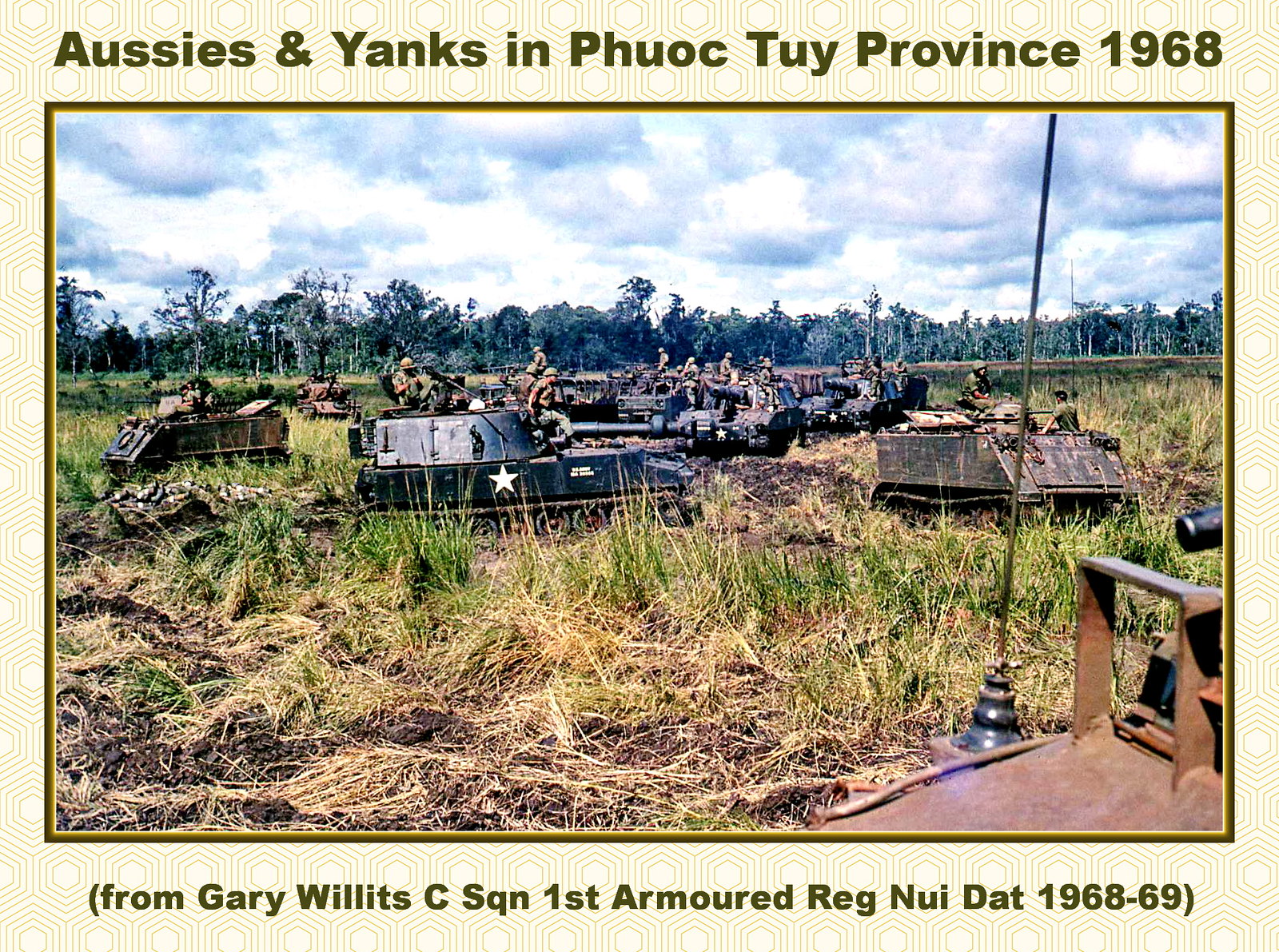The photograph, resembling an image from a history book, captures a historical moment from the Vietnam War. The headline reads, "Aussies and Yanks in Phuoc Tuy Province, 1968," in green. Below, a secondary caption states, "(from Gary Willetts C. SQN, First Armored REG, Nui Dat 1968-69)." The scene is set in a marshy, grassy area with sections of green and dried grass, and is flanked by a backdrop of trees under a blue sky adorned with fluffy clouds. Visible in the foreground are army tanks, some marked with white stars, along with soldiers dressed in green camouflage outfits and helmets. The troops are situated within the tanks and dispersed across the area, though their facial features are indiscernible due to the distance. The overall atmosphere is one of a desolate landscape, marked by the absence of buildings, emphasizing the natural terrain of grass, trees, and open sky.